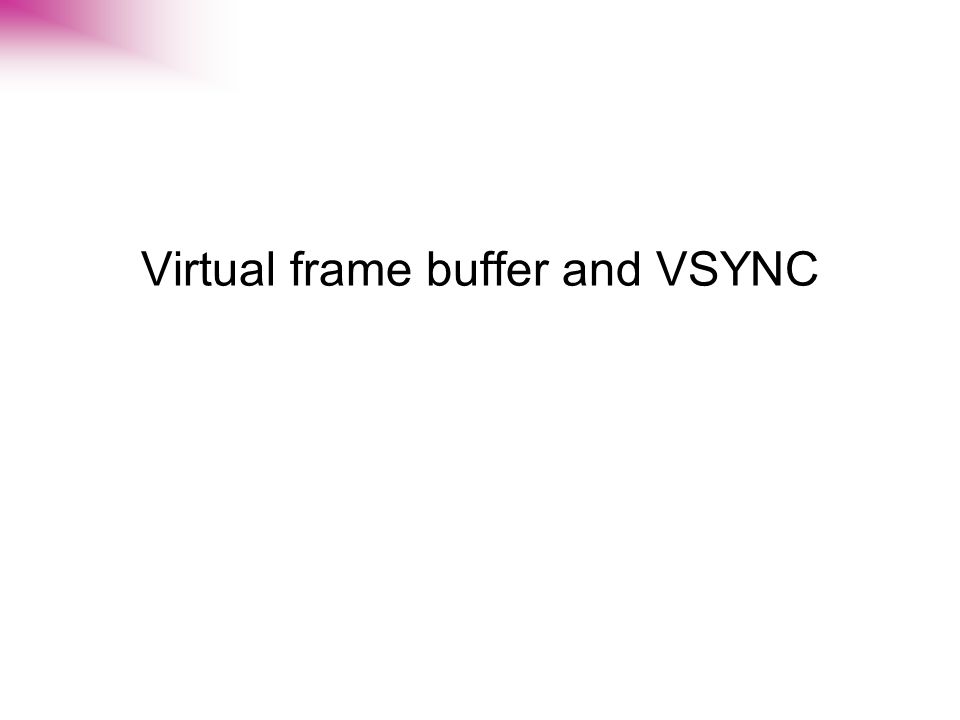The image features a minimalist design typically seen in a display screen or PowerPoint presentation slide. It showcases a white background with a subtle purple gradient blended into the upper left corner. Centered in the image, black text reads "Virtual Frame Buffer" with the acronym "VSYNC" in all capital letters directly beneath it. The image is otherwise dominated by negative space, enhancing the focus on the textual elements. The color palette is primarily white, black, and a hint of purple, making the text the central focus of the graphic.